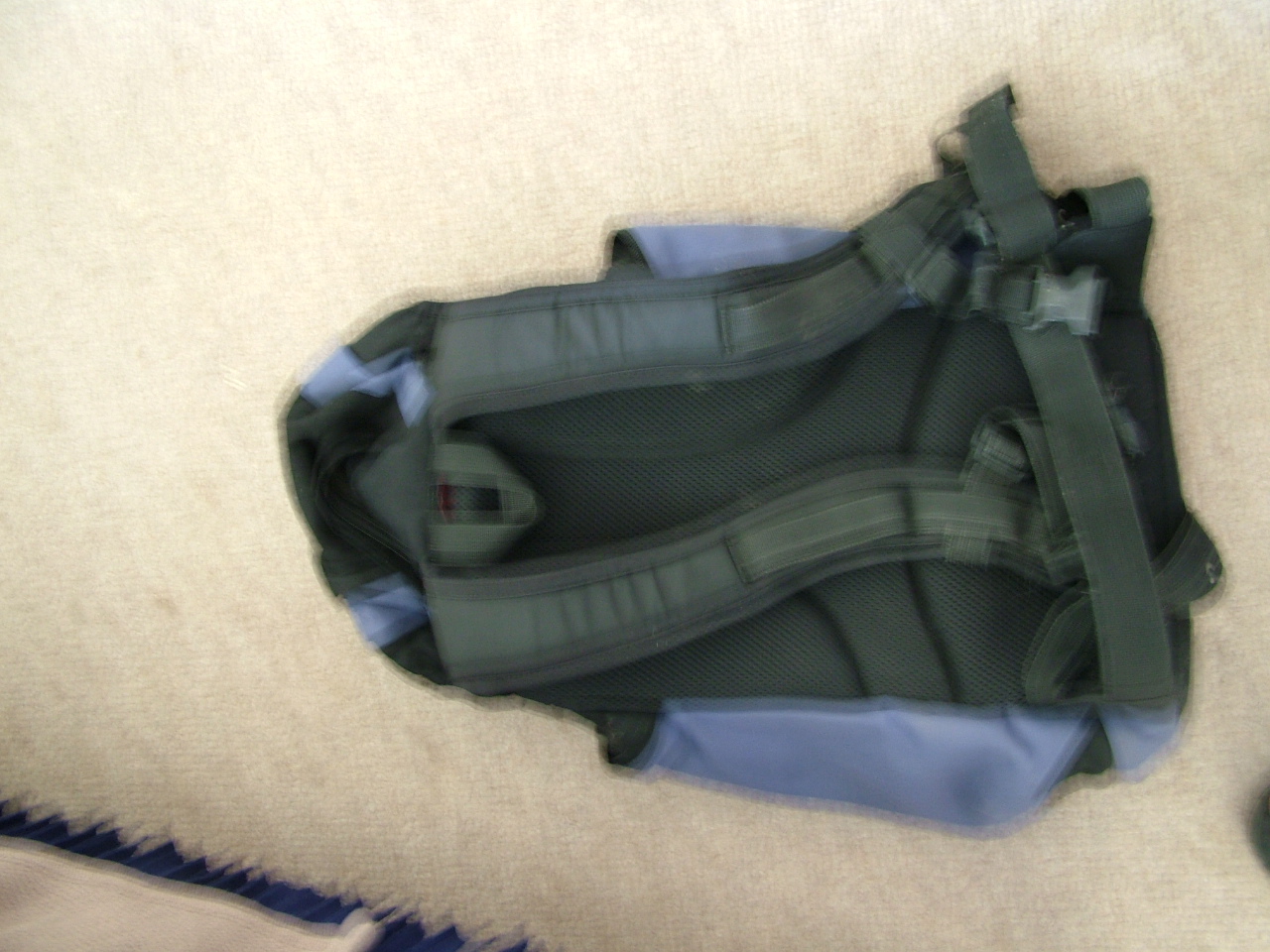The image is a very blurry, out-of-focus picture of a backpack. The backpack is prominently black on the back side, which faces up, with dark bluish sides and top. The backpack features thick, sturdy straps and a utility strap with a hook, suggesting it's designed for heavy-duty use such as hiking or climbing. It has plastic clasps that can secure it around the waist. The setting is indoors, on a beige or cream-colored carpet. Along the bottom left corner, there's a blue carpet with a white cloth or towel draped over it. Additionally, there appears to be a black circular blur in the lower right, possibly a ball. The entire image is very blurry, indicating that it was taken while in motion. The dominant colors and the straps are the most distinguishable features despite the blurriness.